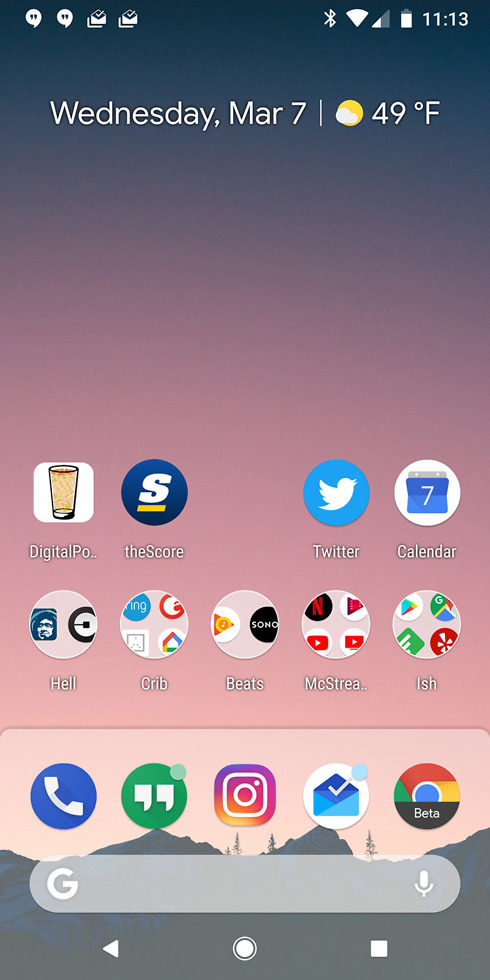The image depicts the front screen of a cell phone. In the upper right corner, there is a nearly full battery icon. Adjacent to it, there's an upside-down triangle and the time displayed as 11:13. Just a couple of inches below, the date is presented in white text: "Wednesday, March 7th." Next to the date, a weather icon shows a sun partially covered by a white cloud with a temperature reading of 49°F.

Several app icons are visible on the screen. There's an app labeled "Digital PO" represented by an image of a glass inside a white square. Another app, "Score," is indicated by the letter "S" in a blue circle. The Twitter app displays the iconic white bird inside a blue circle. The Calendar app shows the number seven in a blue square. Additional apps include "Crib," "Beats," "Mestia," and "Ish," the latter featuring about four different images inside a circle. One notable app, labeled "HELL," features the letters H-E-L-L and an icon of a person with a white face on a dark blue background.

Below these app icons, some quick-access options are visible: a phone icon in a blue circle, two dots in a green circle, and shortcuts for Instagram, Mail, and Google Chrome Beta.